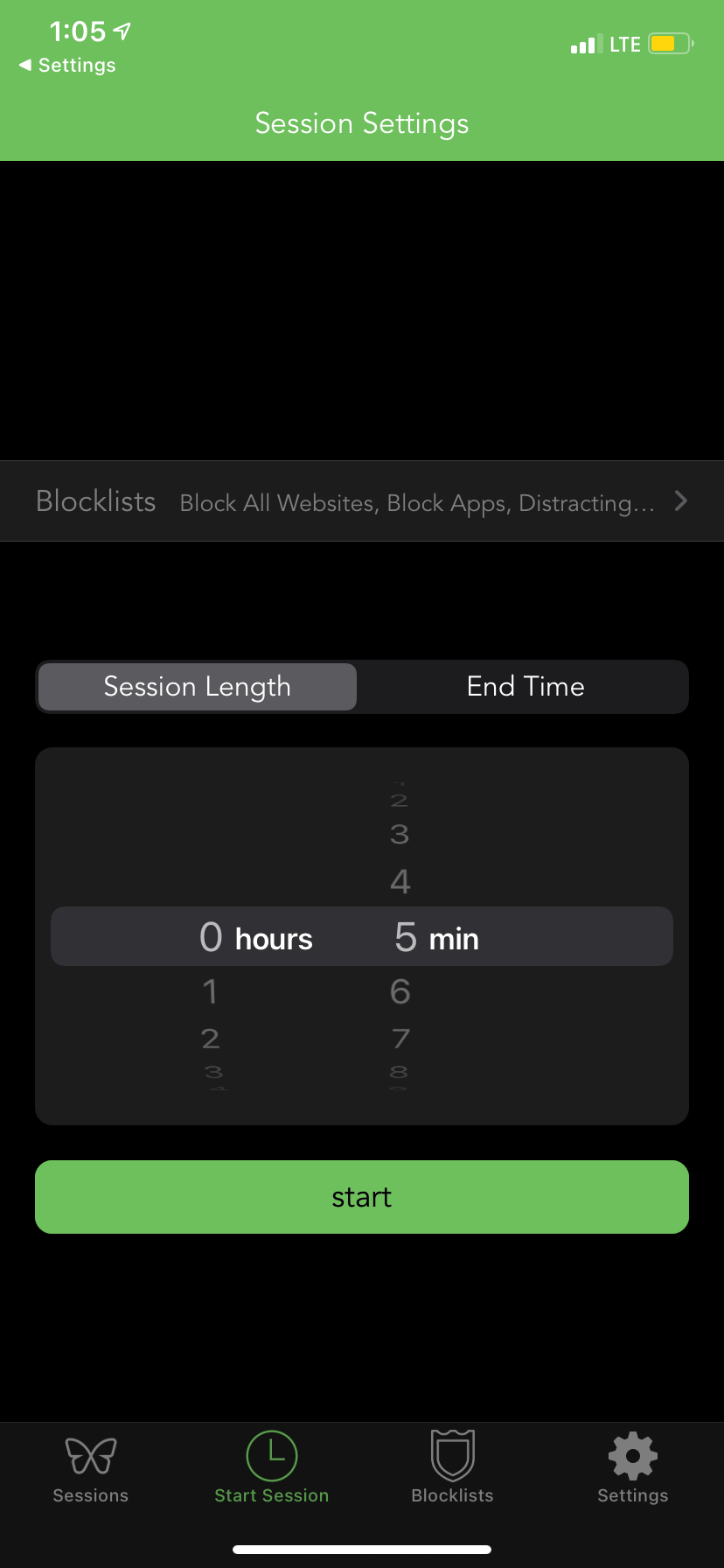The image depicts a screenshot of a digital productivity app interface on a mobile device. At the top of the screen, the device's status bar displays the current time, LTE signal strength, and a yellow battery indicator. 

Directly below, a bold green header with white text reads "Block List." The subsequent section features options for "Block All Websites" and "Block Apps" that are deemed distracting. More settings ensue, including "Session Length," where users can set the desired duration in hours and minutes, and "End Time," also adjustable by hours and minutes. To initiate a session, there is a prominent green button labeled "Start" in black writing.

Lower down the interface are icons representing different sections: a butterfly labeled "Sessions," a clock icon for "Start Sessions," a shield icon for "Block List," and a gear icon for "Settings." The session length option is presented in white text within a gray square, while the end time is shown on a black button with white writing. 

The overall design is sleek and functional, aimed at helping users manage and optimize their productivity sessions effectively.